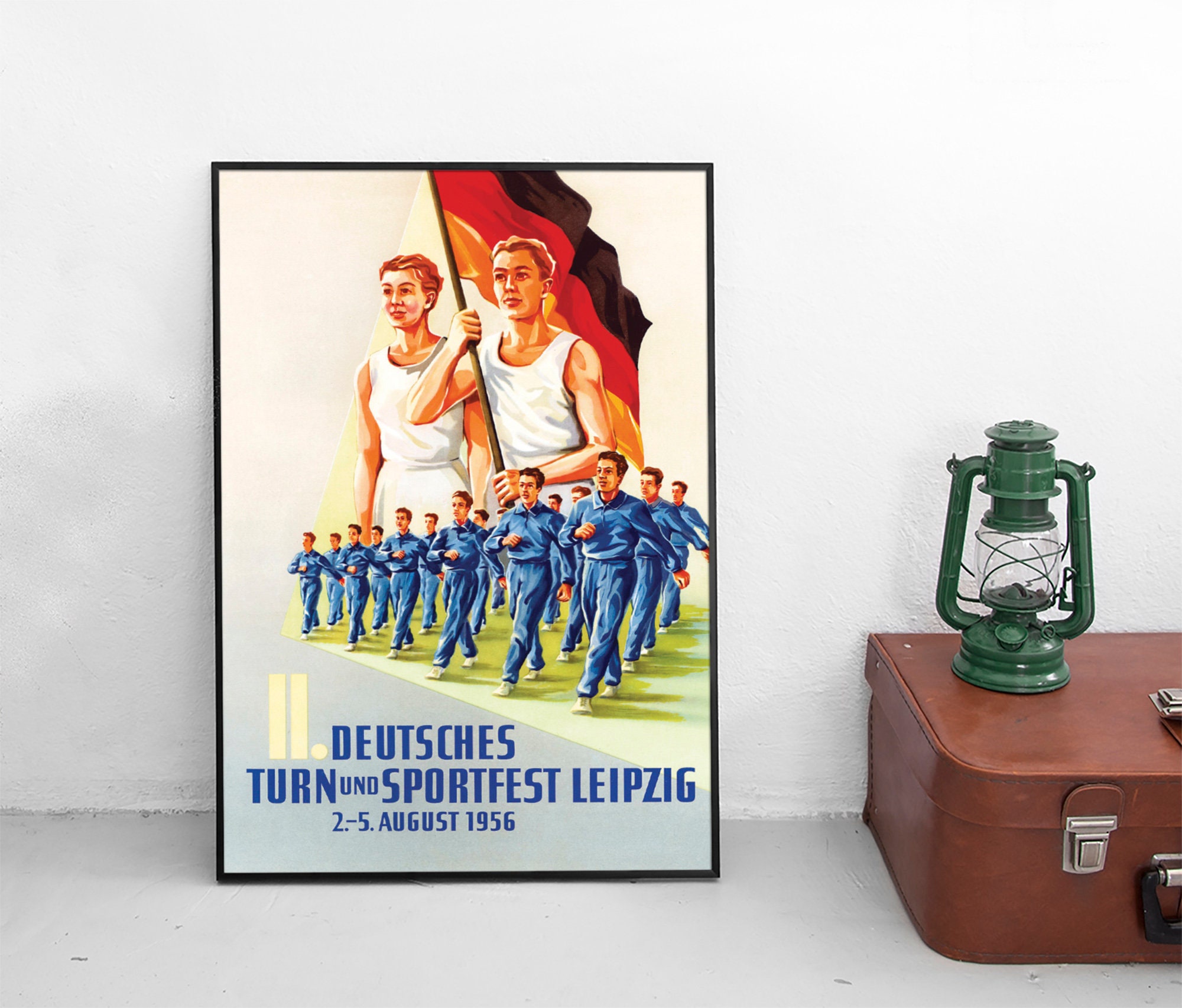The image features a vivid scene captured in a framed poster leaning against a white wall. The poster, encased in a sleek black plastic frame, depicts a sports event dated August 2-5, 1956, labeled "Deutsches Turn-und-Sport-Fest, Leipzig" at the bottom. At the forefront of the image, two blonde-haired women, dressed in white track uniforms consisting of sleeveless tops and shorts, carry the vibrant German flag adorned with black, red, and yellow stripes. Below them, a regimented assembly of individuals dressed in blue track suits, or overalls, stretches or warms up in precise formation, their right arms extending rhythmically across their chests as if in a coordinated march. Adjacent to the poster, on a gray, concrete floor, rests a brown leather suitcase distinguished by a black handle and silver snaps. Atop the suitcase sits an antique green camping lantern, unlit, with a central glass or plastic component that would usually emit light. The composition elegantly juxtaposes elements of athletic history and travel, set against the simplicity of the room's stark décor.